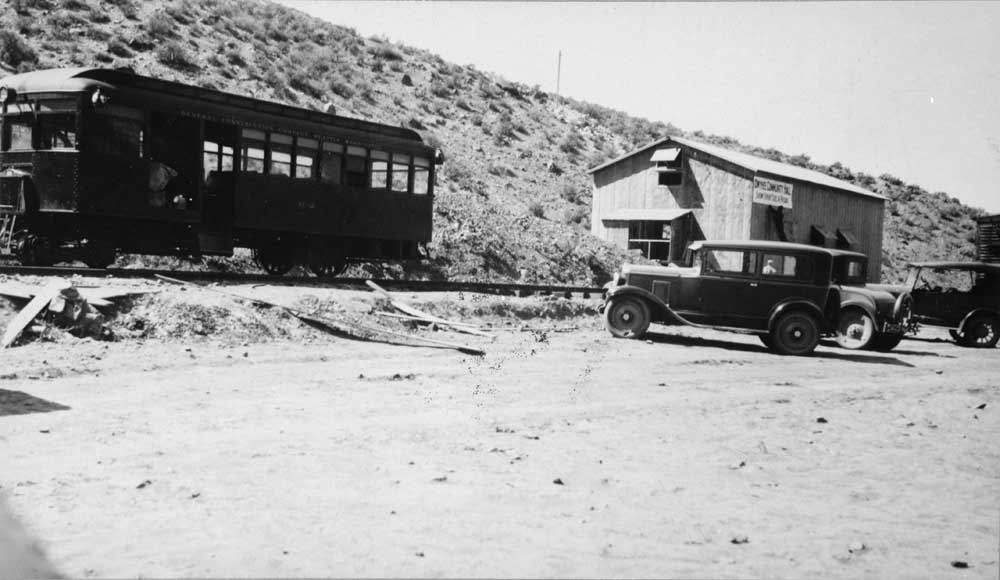This vintage black-and-white photograph captures a scene evocative of the 1930s or 1940s, likely taken somewhere out west. In the image, a lone train car, surrounded by windows and unattached to any other equipment, sits idle on the train track running along the left side. To the right, a small wooden building reminiscent of a barn, possibly an old train station, stands with a sign displaying illegible lettering. In front of the building, three black cars, possibly Model T Fords or vehicles from a similar era, are parked on a dirt road or parking area strewn with rocks and different shades of earth. The background features a hillside covered in sparse scrub and brush, under an expansive, clear gray sky, contributing to the overall dry and rugged atmosphere of the setting.